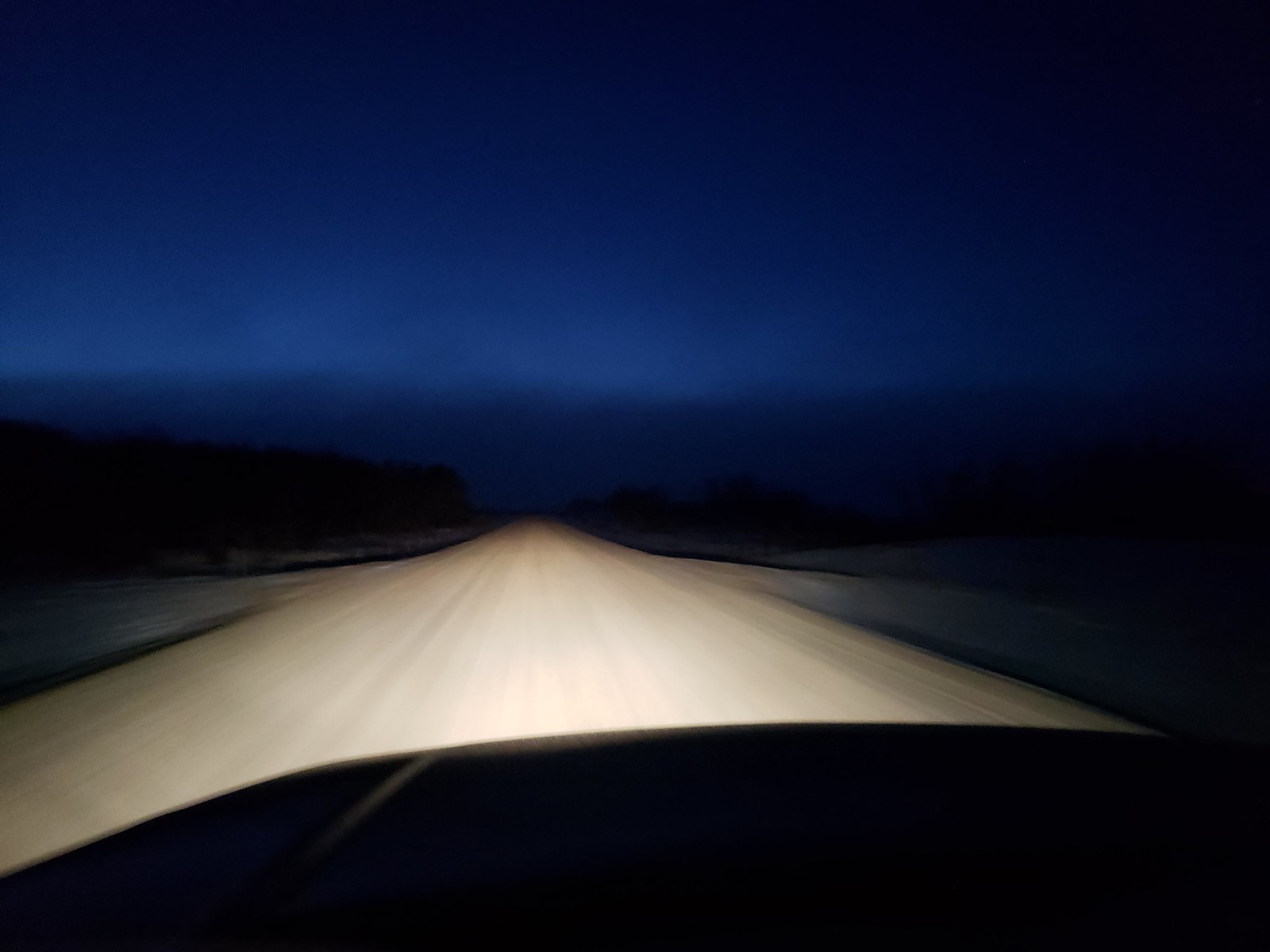This photograph, taken at night from a car, captures the dynamic experience of driving down a remote, dirt road. The image is slightly blurred, suggesting motion as the vehicle travels forward. The headlights brightly illuminate the light brown, beige, and tan road, which features streaks of darker brown and gray. On both sides of the road, mounds of dirt dip and rise, creating a natural border. In the distance, there appears to be a tree line, although it's shrouded in darkness and difficult to discern. The sky above exhibits a gradient of three shades of blue: a deep blue that lightens towards the horizon before merging back into a darker hue. Some faint, blurred hints of white suggest the presence of clouds, though they are barely distinguishable against the night sky. The overall ambience embodies a sense of isolation and mystery, emphasized by the contrasting light and shadows in the scene.